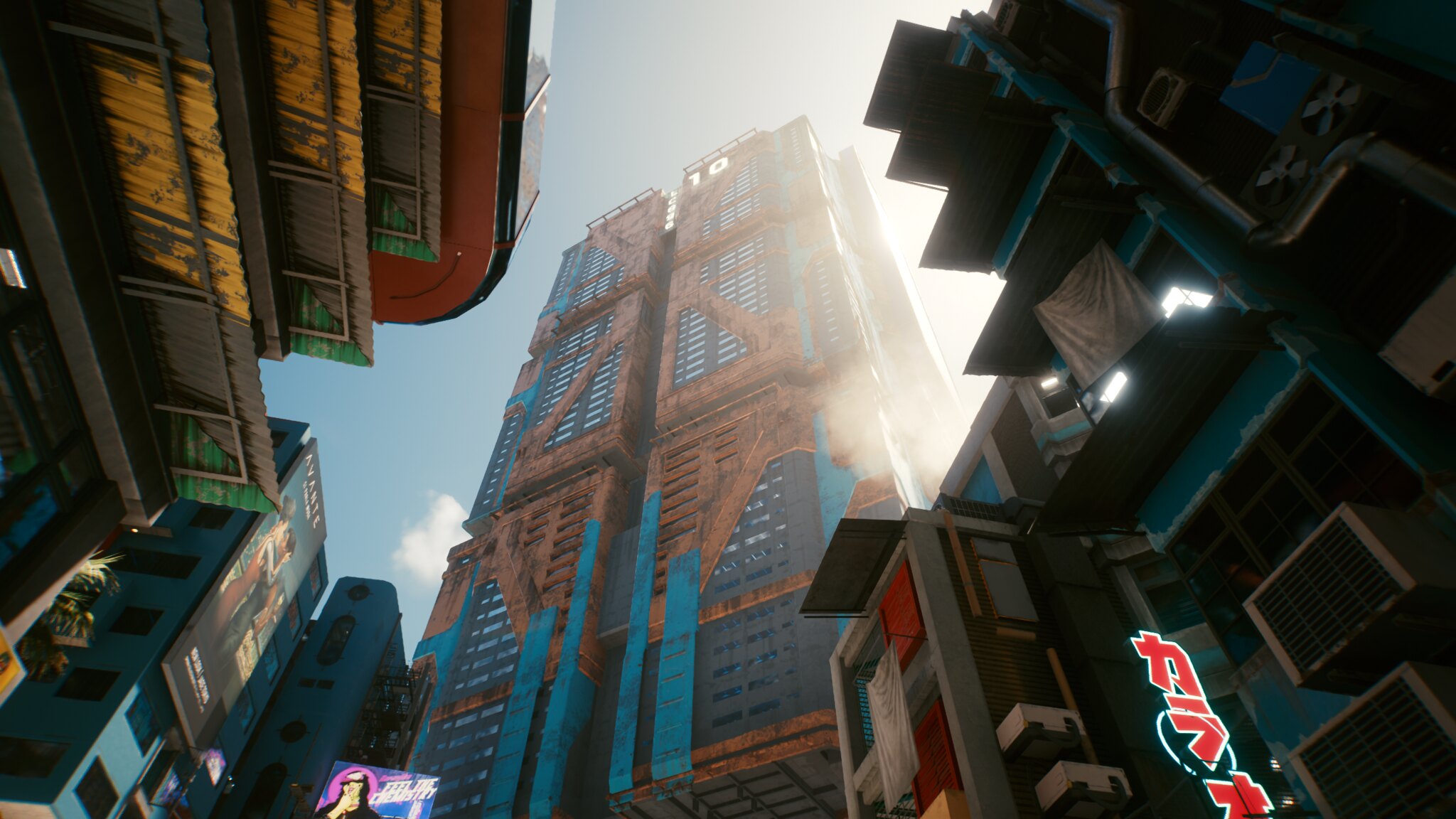This image appears to be a high-quality, detailed rendering from the video game Cyberpunk 2077. The scene is viewed from a street-level perspective, looking up at a series of towering buildings. Dominating the scene is a tall, blue and orange building with narrow windows that might be around 20 to 30 stories high, potentially V's apartment complex from the game. The building's structure includes brown beams crisscrossing its facade, and the number "10" is lit up at the top.

To the left, there is another shorter blue building, while the right side features a blue building that looks like it could be an older apartment complex. This building also sports a neon light in red, displaying Asian script, possibly Japanese kanji.

In front of the taller structures, smaller buildings with an old-style architecture are visible. One of these has a Chinese sign and air conditioners protruding from its side. Balconies extend from each floor, with clothes hanging off one of them, adding to the lived-in feel. The overall aesthetic of the scene combines futuristic elements with a steampunk vibe, showcasing the highly realistic graphics characteristic of Cyberpunk 2077.